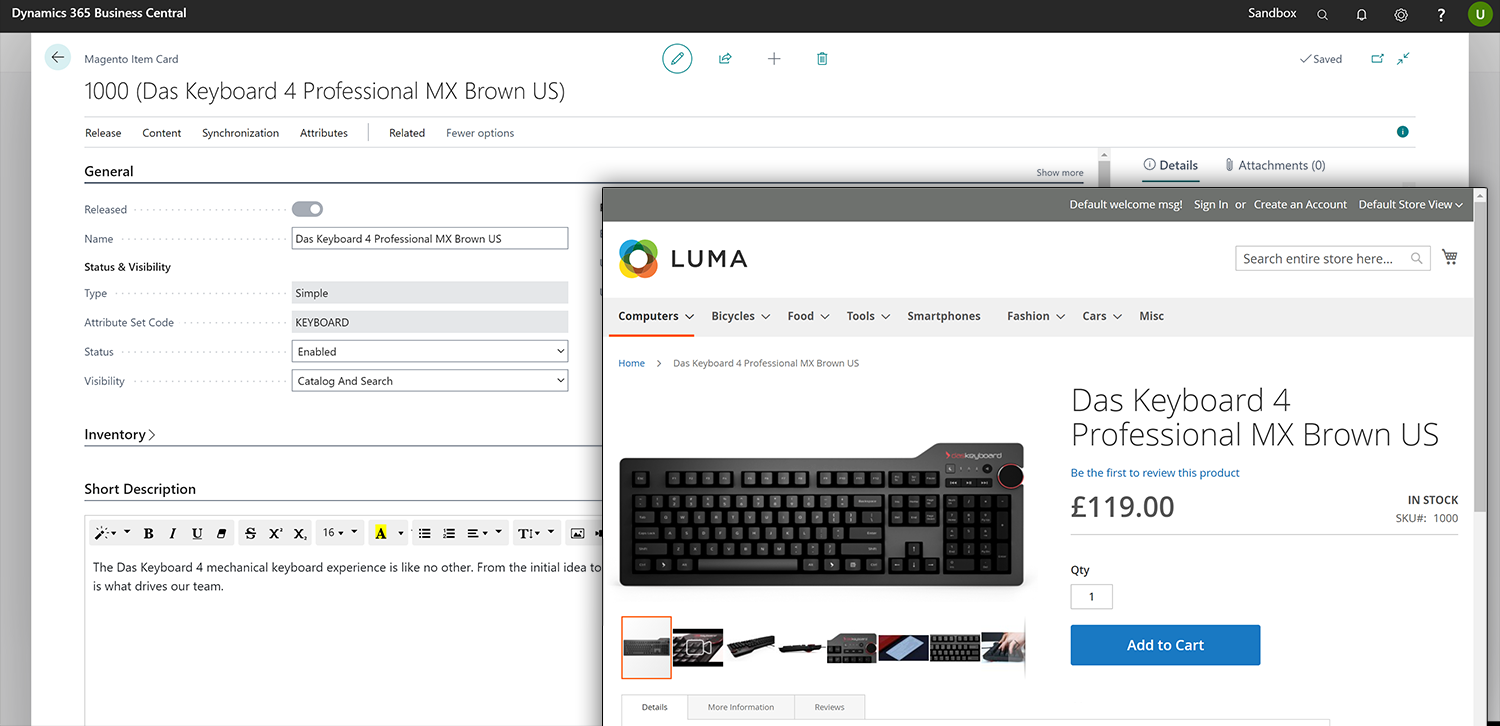This screenshot captures two distinct web pages displayed side by side.

**On the left web page:**
- **Header:** Displayed at the top is a dark grey header with white text on the left side that reads "Dynamics 365 Business Central." To the right of this text is the word "Sandbox" in white, followed by a series of white icons including a magnifying glass, a bell, a cog, and a question mark. On the far right, there is a green circle housing a white capital letter "U."
- **Body:** Beneath the header, the main section of the page is primarily white, flanked by light grey columns on both sides. At the top left of this section is a mint green circle featuring a black arrow pointing left. Adjacent to this, light grey text reads "Magento Item Card." Below that, larger black text displays "1000," followed in parentheses by the description "DOS Keyboard for Professional MX Brown US." The content continues with additional lines of text and various drop-down menus.

**On the right web page:**
- **Header:** This page has a medium grey header. Center-right within the header is white text that says "Default Welcome Msg!" To the right of this message, additional white text reads "sign in or create an account," "default store view," followed by a white downward-pointing arrow.
- **Body:** The main section of the page is white with a color logo on the top left side, composed of overlapping circles in blue, green, orange, and yellow. Centered where the circles intersect is a smaller white circle. To the right of the logo, in all caps, the black text reads "Luma." The rest of the web page content is displayed beneath this header.

This detailed juxtaposition of the two web pages emphasizes the navigation and user interface elements of each clearly.